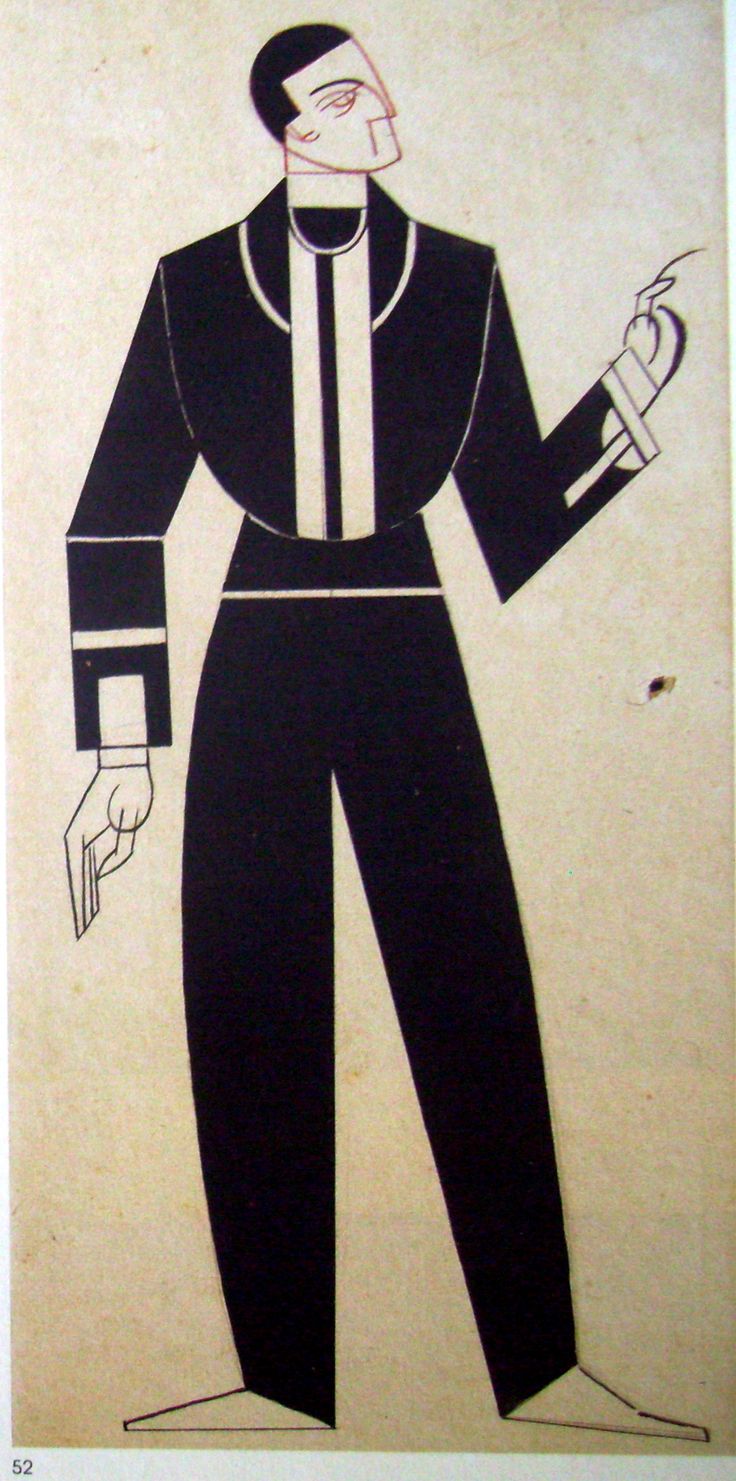This is a vertically aligned rectangular drawing set against a white, paper-like background with faint brown specks. The piece, done in an Art Deco style, features an abstract black and white outline of a man. His figure is filled predominantly in black, with strategic white accents. His head, rendered in white and detailed minimally with one visible eye, a nose, a hint of an ear, and black hair, faces the right. However, his body is oriented towards the viewer. The man appears to wear a stylized tuxedo, comprised of a black jacket with two vertical white lines descending from his collar to his waist, which is delineated by a thin horizontal white stripe. His right arm, slightly bent, hangs down with the palm facing towards his right leg. The left arm is bent at the elbow, with the forefinger pointed up towards the left side of the image. His feet aren't clearly defined but are represented as triangular shapes pointing outward.